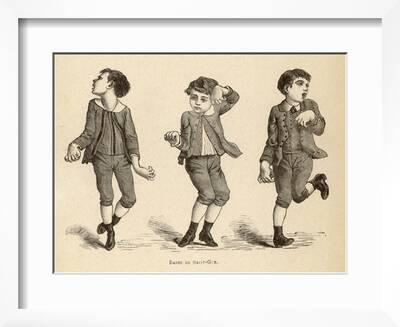The framed picture features a vintage illustration of three young boys, around seven or eight years old, dancing joyfully. Encased in a white matting and a silvery, possibly white wooden frame, the artwork exudes an old-fashioned charm, reminiscent of the 1920s or 30s. The image is rendered in sepia tones with shades of beige, black, gray, and white, giving it a nostalgic feel.

The boys are dressed in period-specific clothing, including capri-like knickers paired with socks that meet the knickers' ends, black leather boots, and one of them sports a vest, jacket, and tie. Each boy strikes a unique dance pose: the boy on the right lifts one leg and holds one arm closer to his chest while looking towards the top right. The middle boy raises one arm above his head and holds the other wide, his gaze directed downward. The boy on the left crosses one foot behind the other with both arms extended and looks toward the top left. Their shadows cast beneath them add depth to the lively scene, capturing a moment of carefree exuberance.